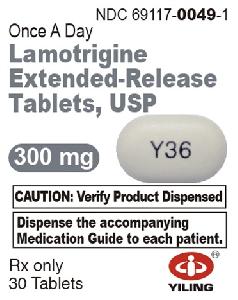**Description Caption:**

This image appears to be a detailed portion of a medication packaging for Lamotrigine Extended Release Tablets, USP. The top right corner displays the National Drug Code (NDC) number "NDC 69111/0049/1," with "0049" bolded for emphasis. On the left-hand side, the text reads "One a day Lamotrigine Extended Release Tablets, USP." Just beneath this text is a small grey rectangle with curved edges, containing "300 milligrams" written in white text. 

On the right side of the image, there is a 3D-rendered depiction of one of the tablets, which is grey in color and imprinted with "Y36" in black text. Below the pill image, there are two prominent black boxes with bolded text: the first reads "CAUTION: Verify product dispensed," and the second states "Dispense the accompanying Medication Guide to each patient". 

At the bottom of the image, either on the right or left corner (exact positioning unclear), "RX Only, 30 Tablets" is printed, indicating prescription-only status and the tablet count. Additionally, there is a grey oval icon with an "i" in the middle, encircled by two bands that resemble a stylized person with their head and arms extended, accompanied by the text "Wiling" written in black. 

Given the details, this image likely represents a section from the packaging of Lamotrigine, a medication used as an anticonvulsant, rather than an internet advertisement.